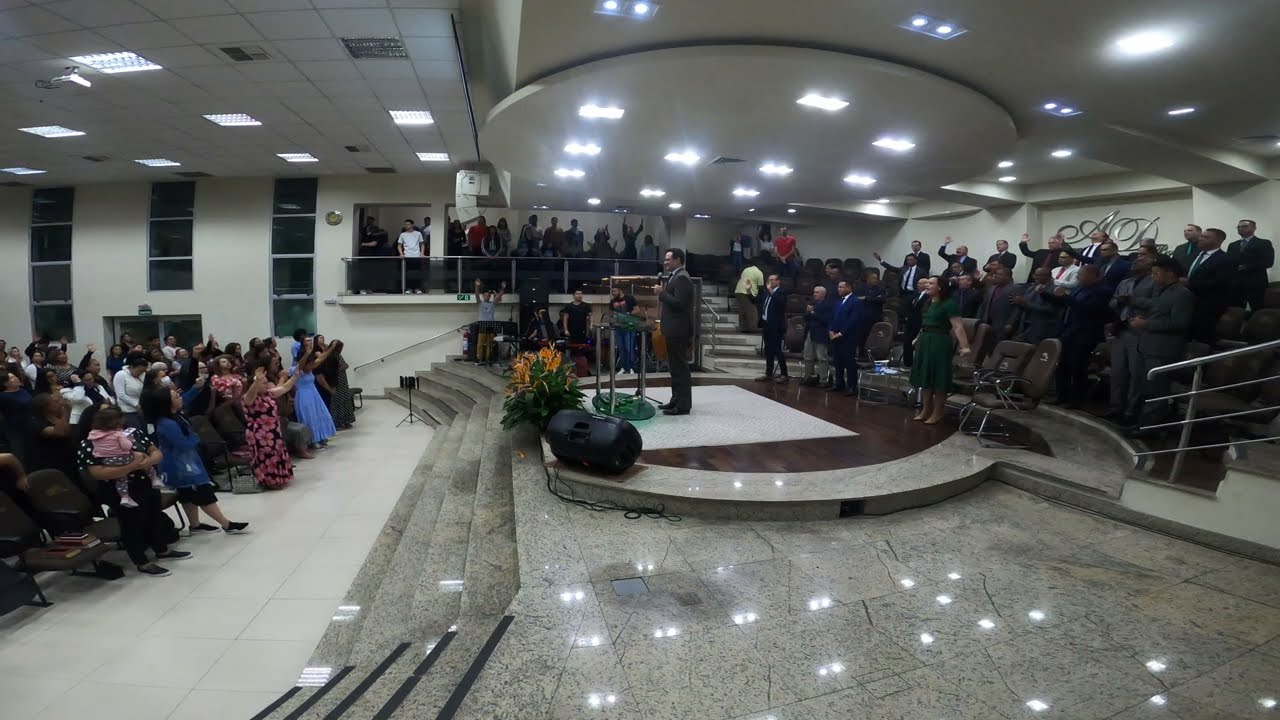This image captures a large, indoor church gathering, prominently featuring a speaker standing at a gray granite podium in the center of the assembly. The setting is a spacious venue with a tall, white ceiling adorned with lights that reflect off the shiny floor. The congregation is dressed formally; women are in long dresses while men don suits and ties. The speaker at the podium, a man in a suit holding a microphone, addresses a mixed audience. In front of the podium is a planter with vibrant orange flowers. Surrounding him are men in suits seated on chairs, possibly a choir, although not in traditional choir attire. Additional attendees are positioned on a balcony to the right of the speaker, involving a few steps up, watching and participating in the proceedings. Many people, both seated and standing, have their arms raised, contributing to the dynamic atmosphere of the gathering.